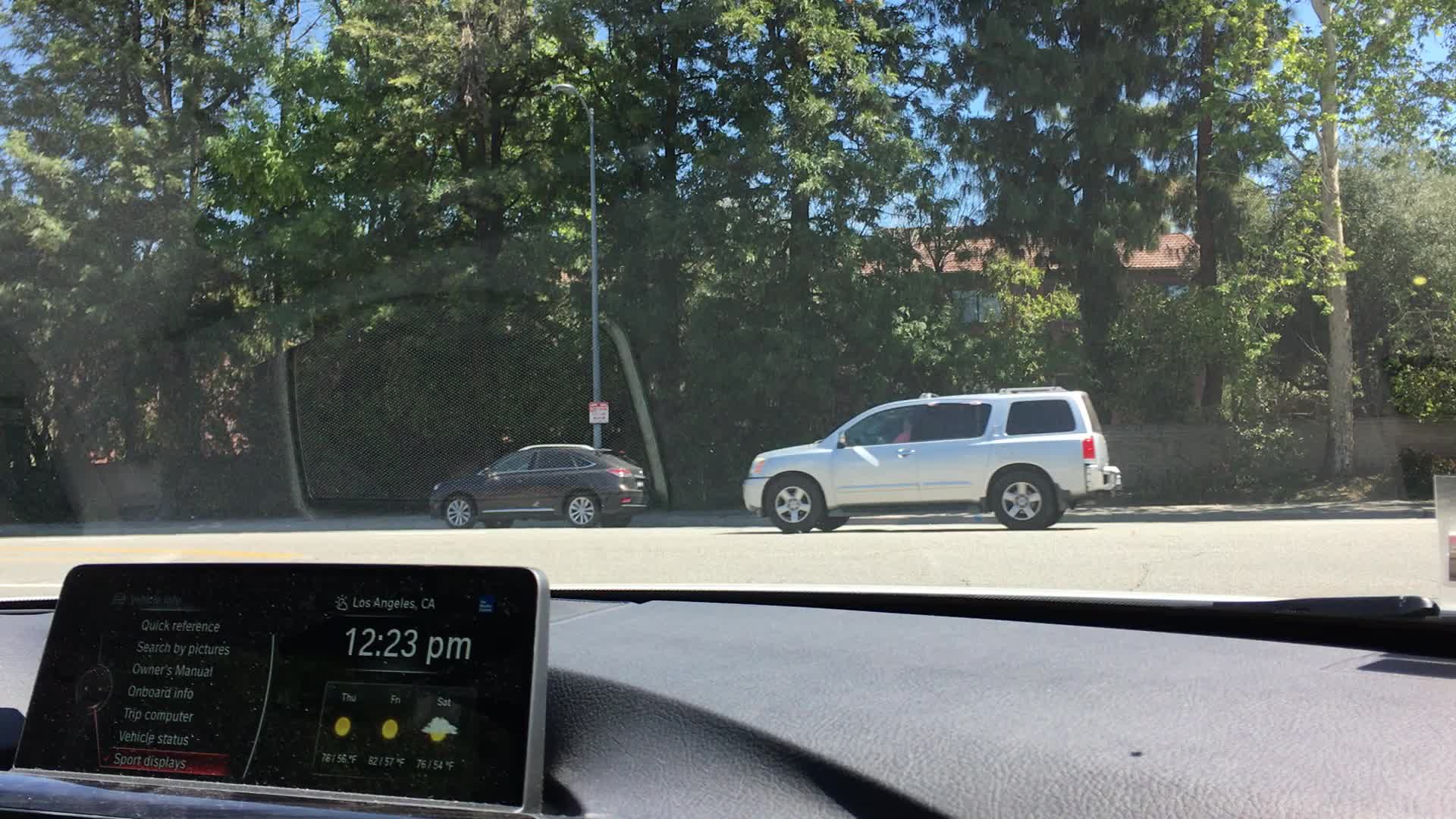This is a color photograph taken from inside a car positioned at an intersection or waiting to pull out onto a busy road. The interior view reveals a gray dashboard with a small digital screen displaying various commands on the left side, including an "Owner's Manual" and "My Computer." The right side of the screen shows the time as 12:23 PM and presents the weather forecast for Thursday, Friday, and Saturday, with visible icons of suns and clouds. You can also see the bottom of a windshield wiper.

In the scene beyond the windshield, bathed in sunlight under a blue sky with some shadows, there are two vehicles traveling from right to left. The first is a compact, burgundy-maroon car, possibly a coupe, and the second is a very large, white SUV with tinted windows. Behind these vehicles, a tree line composed of various deciduous trees with their leaves on is visible. A small, red-roofed brick house peeks through the trees, and a solitary street light stands with a white and red sign attached. Additionally, there appears to be a short brick wall near the SUV. The landscape and the road indicate an outdoor suburban setting in America.